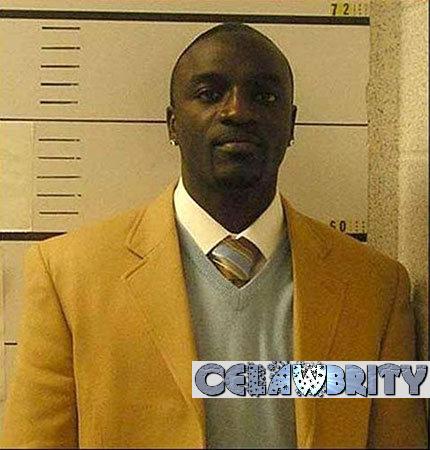The image depicts a black man with very short black hair and a small goatee. He has earrings in each ear that appear to be diamond-like. He's dressed in a white shirt, topped with a blue vest, and a blue and yellow tie. Over this ensemble, he wears a mustard-colored suit jacket. The background is white with a prominent black line near the top, clearly marked with the number '72' and '60' just above his left shoulder. This black line is accompanied by smaller lines beneath it, likely for measurement. There's also a banner with the stylized text "C-E-L-A-W-B-R-I-T-Y" in blue with a black border, resembling a unique, almost shimmery font. The man’s expression is calm, with a slight, understated smile.